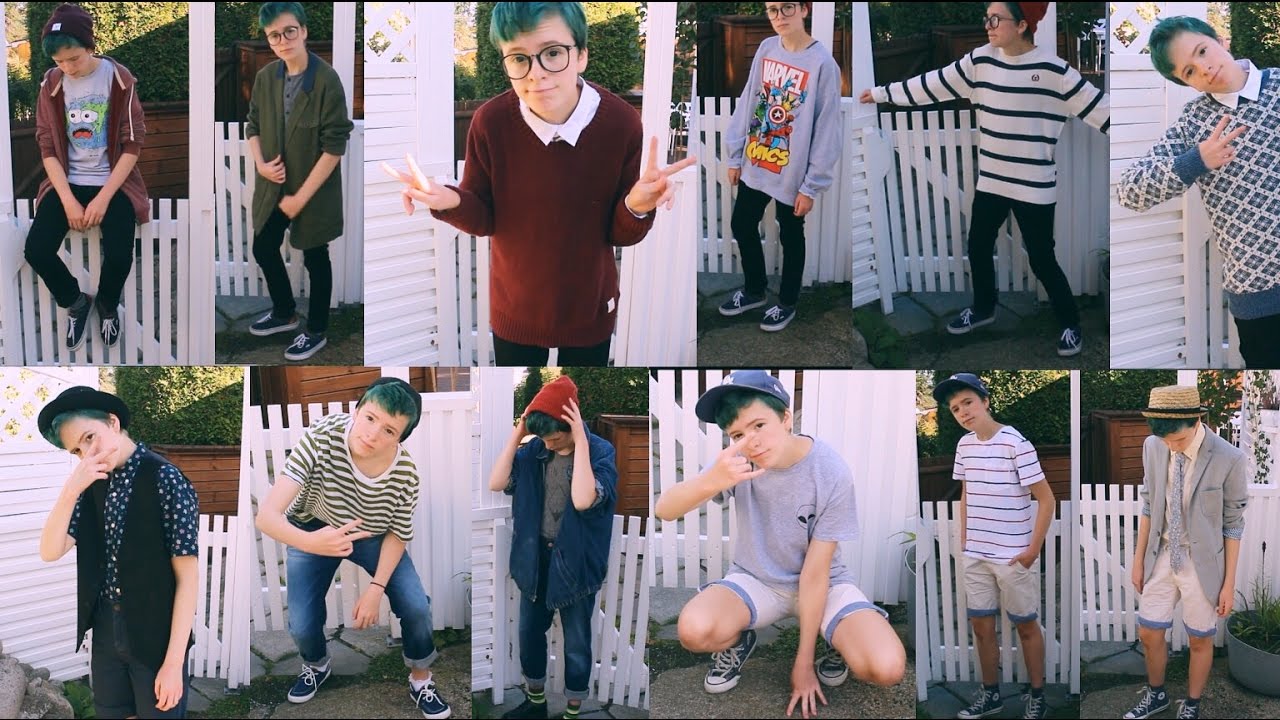This is a collage comprising twelve photographs arranged side-by-side in two rows of six. The images feature a pale-skinned, eight-year-old boy with striking hair that appears green in some photos and blue in others, suggesting either different lighting or dye variations. Most notably, he has short hair and wears thin-rimmed black glasses in four adjacent photos in the top row.

Each photograph showcases the boy outdoors, likely in a backyard setting, with a white picket fence and natural foliage visible in the background, alongside a brown building in some shots. The boy engages in various poses, including making a peace sign, spreading his arms, squatting, and forming a heart with his hands.

The boy's outfits are diverse and carefully styled, including a combination of casual and playful attire. He sports items such as a beanie and Cookie Monster shirt, a Marvel Comics T-shirt, striped and short-sleeved shirts, jeans, khaki and white shorts, Converse shoes, a long jacket, a vest, a blue shirt, a jean jacket, and even formal wear with a suit jacket, tie, and straw hat. Each image captures a unique facet of his wardrobe and personality, encapsulating a vibrant and varied display.